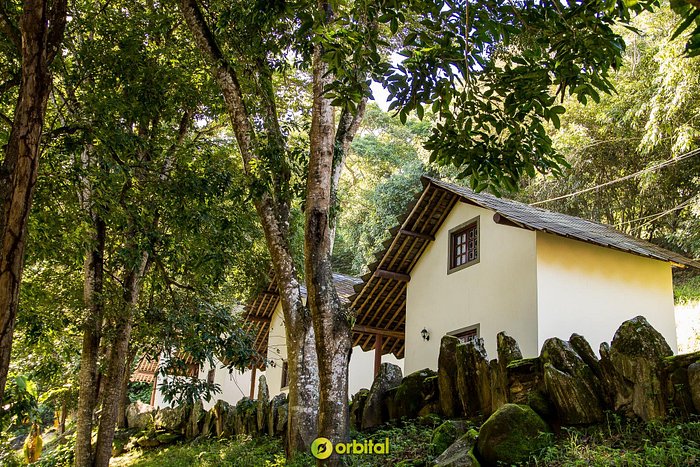This photograph depicts a small, rustic house or cottage, set amid an abundance of greenery, indicative of a warm climate. The house, constructed from white stucco with a dark brown, sloping wooden roof, features a single upper-floor window and a front doorway adorned with a porch light. The scene is set against a backdrop of tall trees and dense foliage, suggesting a forest beyond the property. Surrounding the house is a primitive, uneven fence made from rocks and wood, contributing to the rustic charm of the setting. The foreground presents lush green grass and a glimpse of a clear, sunny sky. To the left, partially obscured, are additional similar cottages, hinting at a collection of identical structures, possibly part of a quaint, countryside hotel or residential area. At the bottom center of the image, the brand name "Orbital" is displayed in yellow font beside a yellow circle logo, which might resemble an acorn. The overall composition and bright daylight suggest a serene, summery atmosphere, reminiscent of picturesque Swiss chalets.